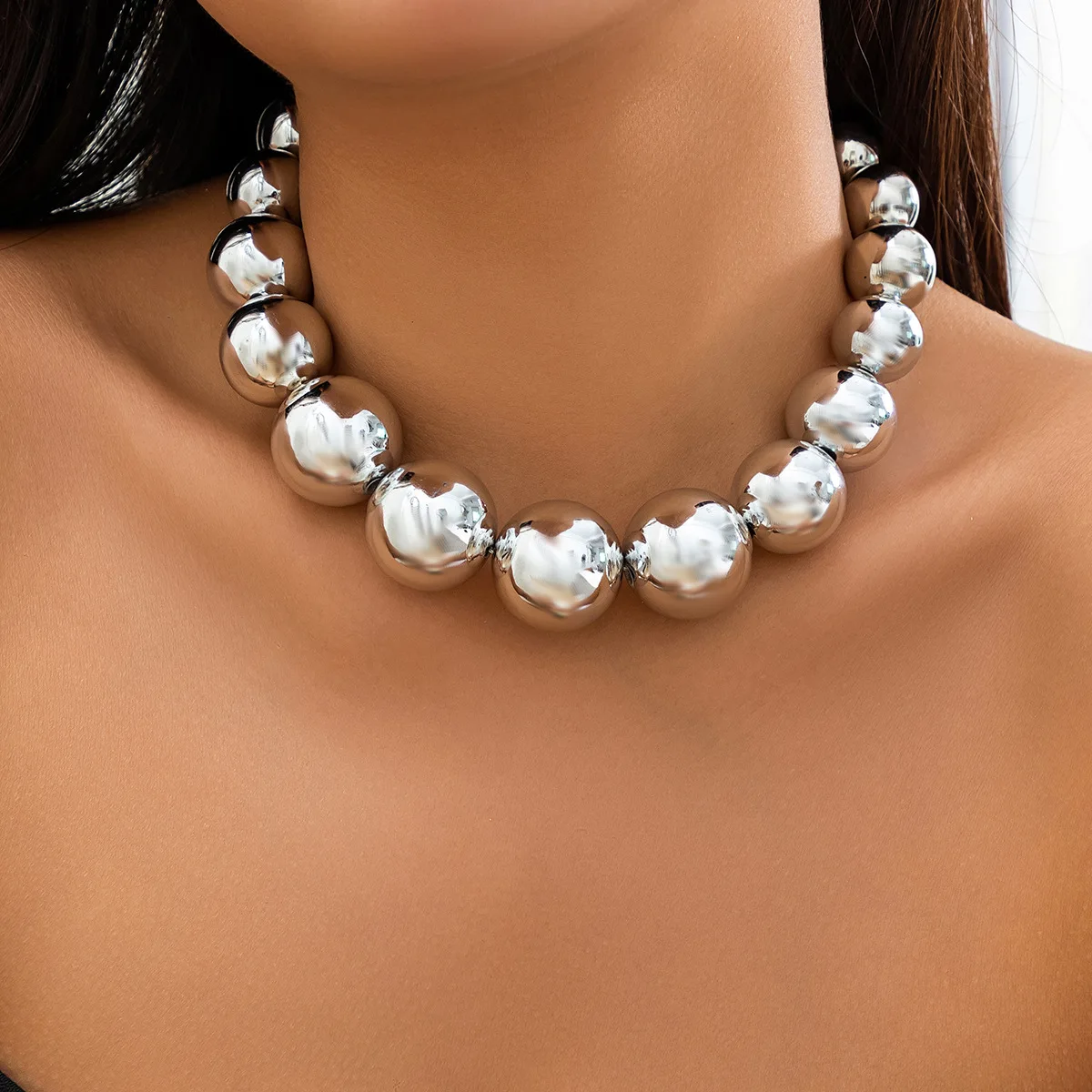This is a professionally styled, close-up image capturing the neck and collarbone area of a woman with fairly tanned, possibly olive-toned skin. The lower portion of her chin and the long, straight strands of her dark brown hair are also visible at the top of the image. She is standing against a white background, lending clarity to the primary focus of the image: her necklace. The necklace, composed of approximately 15 large, shiny silver beads, each about 1 to 1.5 centimeters in diameter, drapes elegantly along her neck. The beads' smooth surfaces reflect light, emphasizing their glossy finish and adding an element of sophistication to the composition.